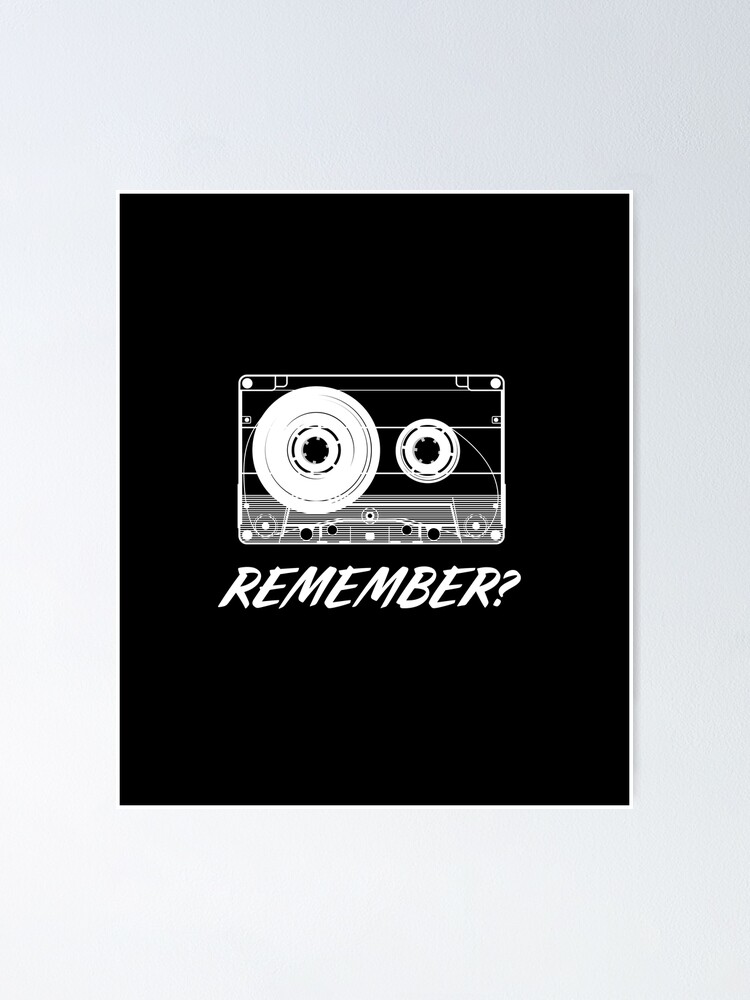The image depicts a digital artwork hanging on a white wall. The centerpiece of this artwork is a black square with a thin white outline, subtly accentuated by a gray drop shadow, suggesting a framed presentation. The focal point within the black square is a detailed, white line drawing of an old cassette tape. This tape features two spindles: the left spindle is densely wound with tape, while the right spindle appears almost empty, connected by a thin strip of tape. The tape, rendered with such precision, even shows the small circles or holes where it would fit into a player. Below the cassette drawing is bold, white text resembling handwriting or perhaps a marker font, which reads "REMEMBER?" in all capital letters. The background of the overall image is a light gray, almost white, enhancing the contrast and making the black square and its contents stand out prominently.